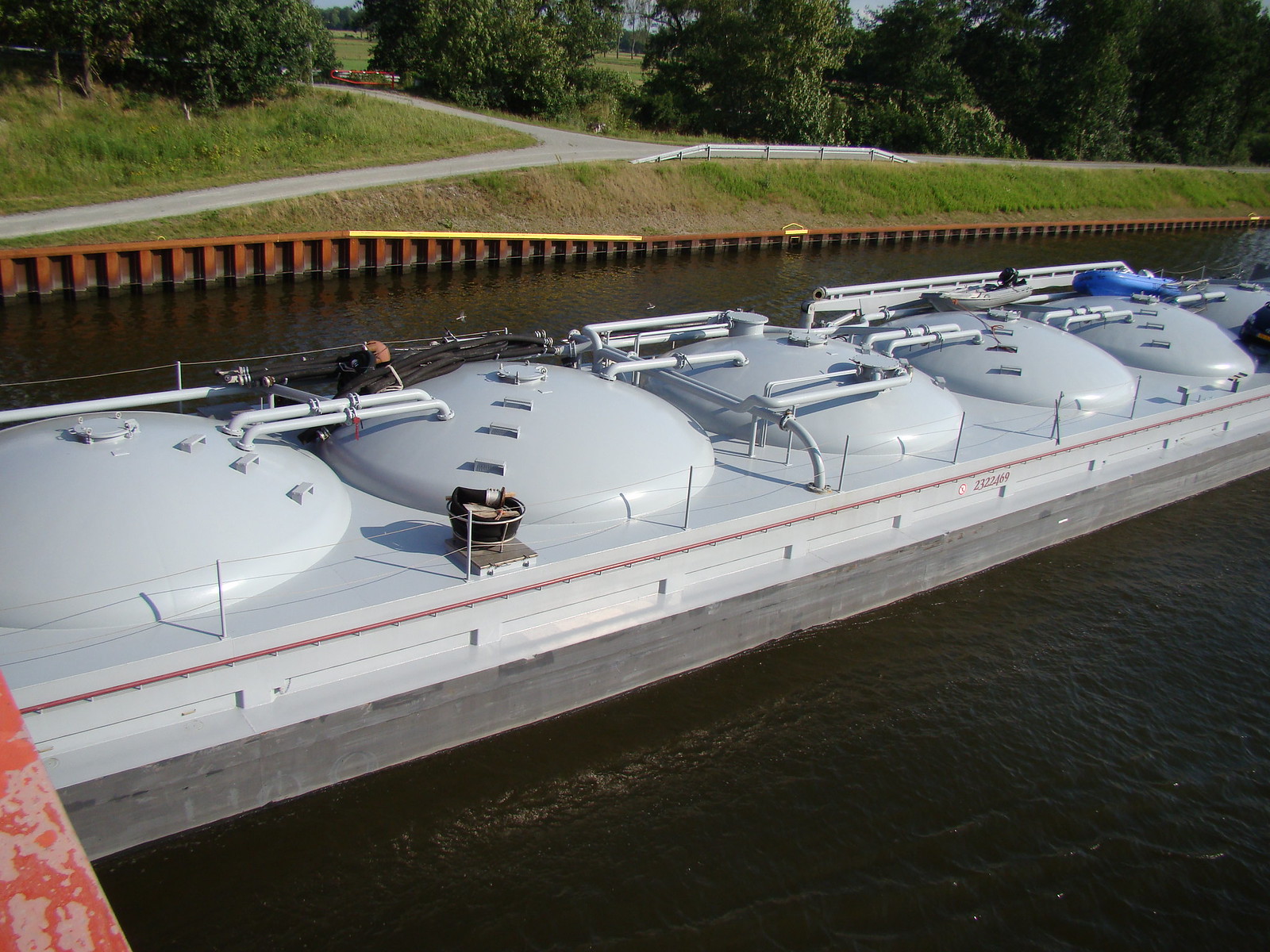This image showcases a large, rectangular, floating structure resting on dark, brownish-black water, possibly a lake or pond. The structure appears to be constructed from gray metal and wood, resembling a segment of a pipeline or an industrial platform, with several visible gray pipes and tubing. It has five or six prominent, circular, bulbous tops interconnected by piping and fitted with railings and handholds. The backdrop features a grassy, hilly area with a narrow, desolate roadway meandering through it, flanked by green fields or pastures. Further in the background, dark-colored trees and dense shrubbery create a natural border. Additionally, a red and pink object is noticeable at the bottom left corner of the image. The photo presents a landscape view with the structure positioned diagonally from left to right.